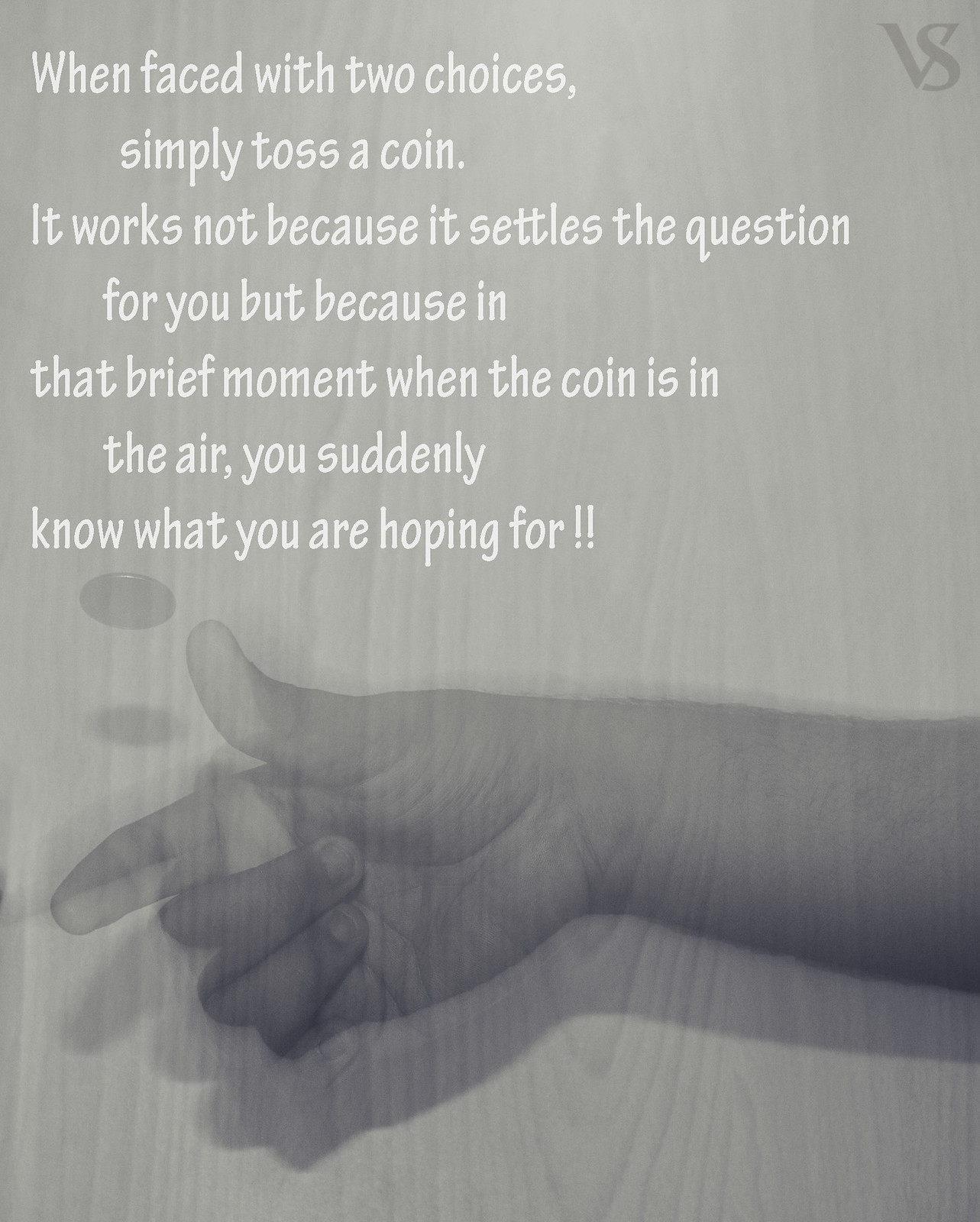The image shows a motivational poster with a slight wood grain background. Dominating the bottom third of the image is a child's hand with four visible fingers—the thumb, index, and middle fingers extended, while the pinky and fourth finger bend into the palm, possibly clutching something. This detail creates the impression of flipping a coin, though no coin is visible. The text at the top, spread across seven lines and followed by two exclamation marks, reads: "When faced with two choices, simply toss a coin. It works not because it settles the question for you, but because in that brief moment when the coin is in the air, you suddenly know what you are hoping for." Additionally, the letters "VS" in light gray are placed at the top right corner. The overall tone of the image aligns with content typically shared on social media or used in motivational contexts.